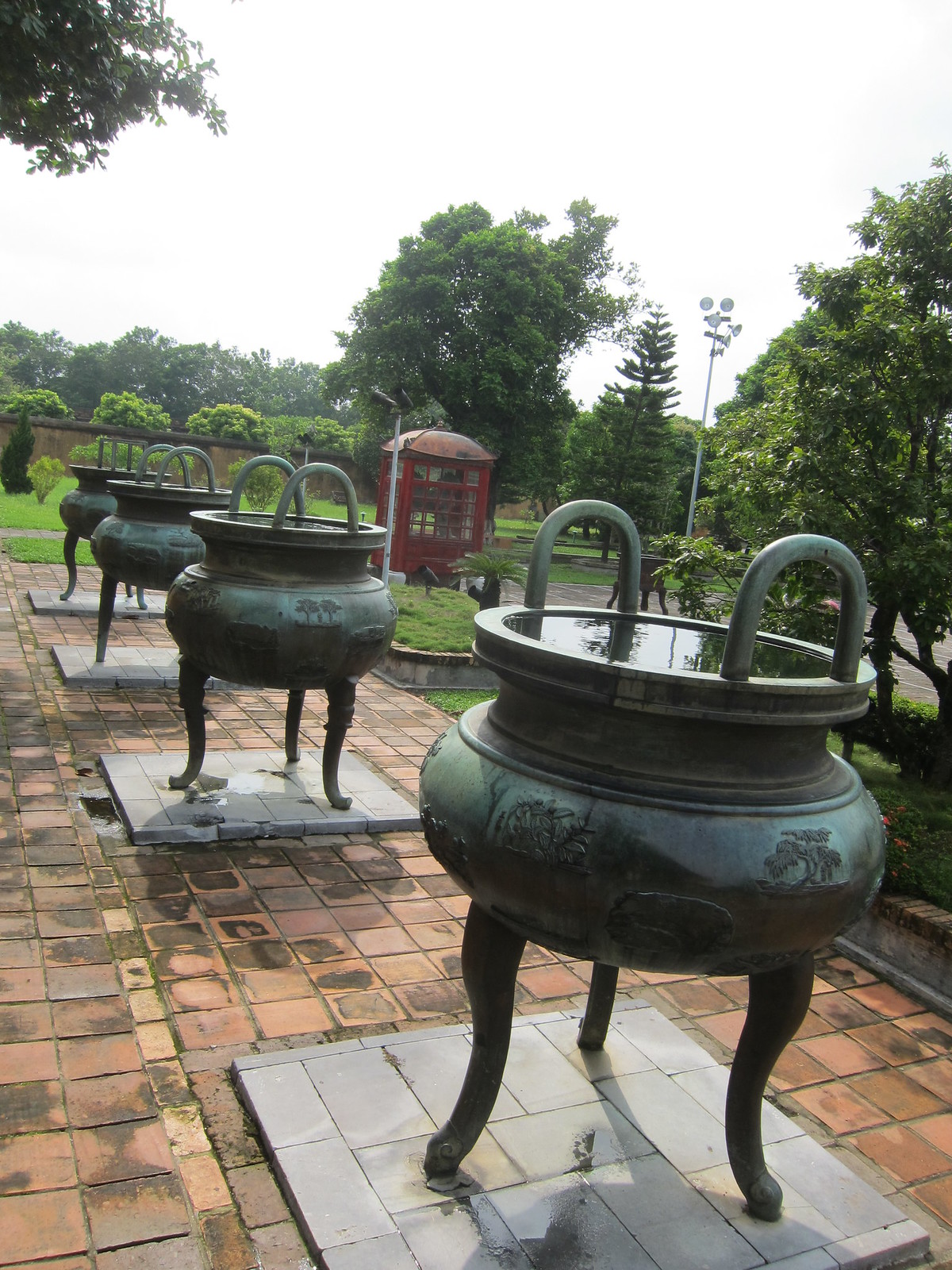This photograph captures an exquisite scene of four massive bronze or copper dynastic urns, identified as national treasures from the Hue Imperial Citadel in Vietnam. These urns, aged to a greenish-brown patina, stand proudly on a slate-raised platform composed of gray bricks, which itself is placed on a paved walkway of red square bricks. Each urn is elevated on three curved legs and features intricate carvings—likely depicting trees—encircling their bodies. The urns also boast large ridged rims with two substantial hoop handles extending upwards.

The setting is reminiscent of an English garden, with a backdrop of lush green grass, verdant trees, and bushes lining a tall wooden fence. A red, somewhat tarnished telephone booth-like structure with a black roof and window panes sits towards the back, adding a quaint charm. Brown brick pathways lead through the scene, and a white pole with multiple lights, perhaps for illumination and security, looms in the background under a gray, overcast sky.

The garden is vibrant, with well-maintained greenery, and it appears that it has recently rained, as evidenced by the wet pavers. The overall ambiance of the photograph is serene and historical, seamlessly blending natural beauty with ancient artifacts.